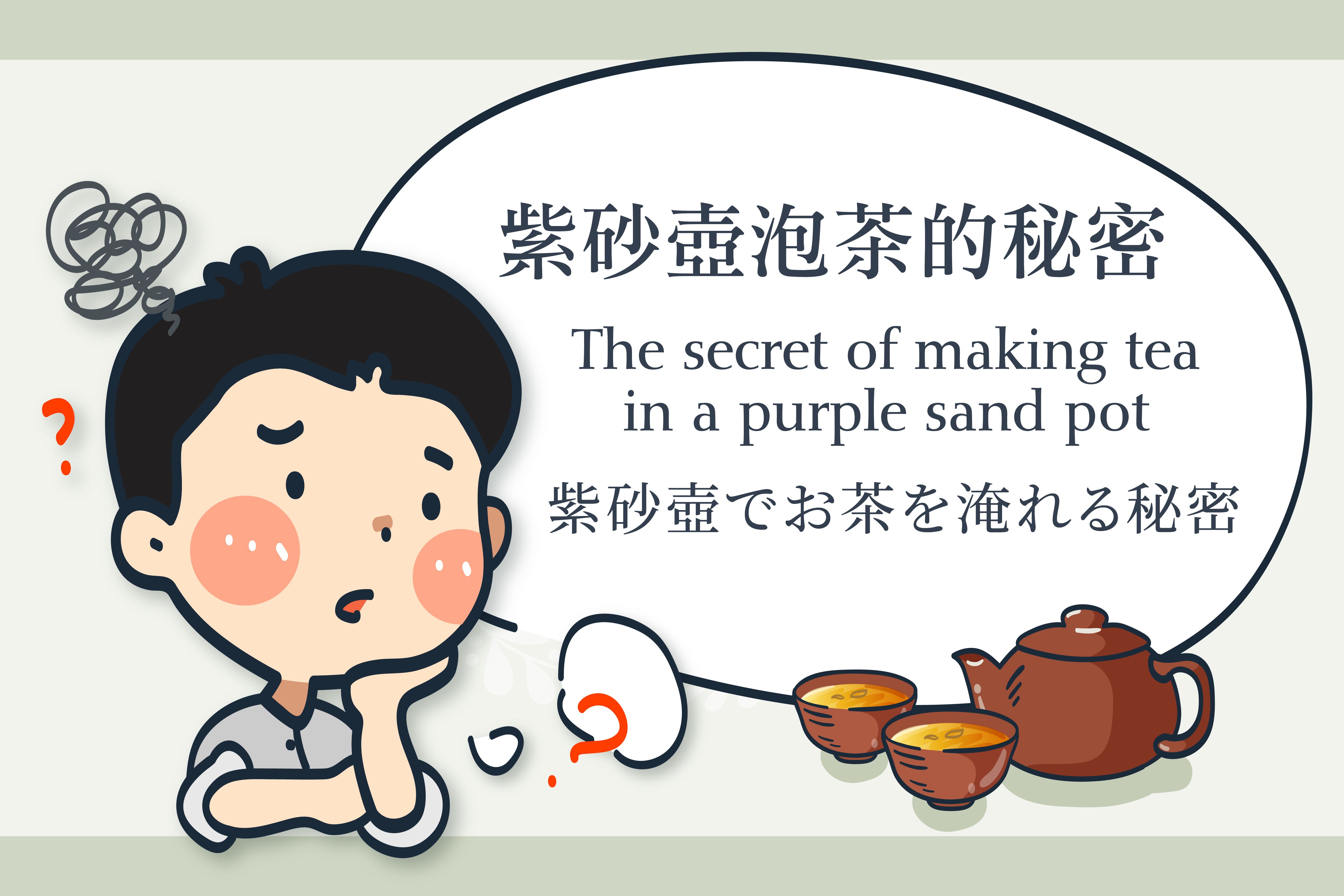The detailed cartoon image features an advertisement, likely Chinese, and centers on a young boy in a white button-up shirt with rolled-up sleeves. The boy, with dark, cartoonish hair, blush-streaked cheeks, and a quizzical expression, is depicted in deep thought, resting his chin on his left hand. Behind him, there are squiggly lines, red question marks, and a black thought bubble, enhancing his contemplative demeanor. The prominent English text, "The Secret of Making Tea in a Purple Sand Pot," dominates the right side of the image, surrounded by Chinese characters. Below the text, there's an illustration of a reddish-brown teapot accompanied by two matching teacups filled with yellow tea. This vibrant, comic-like scene emphasizes the intriguing process of traditional tea-making.